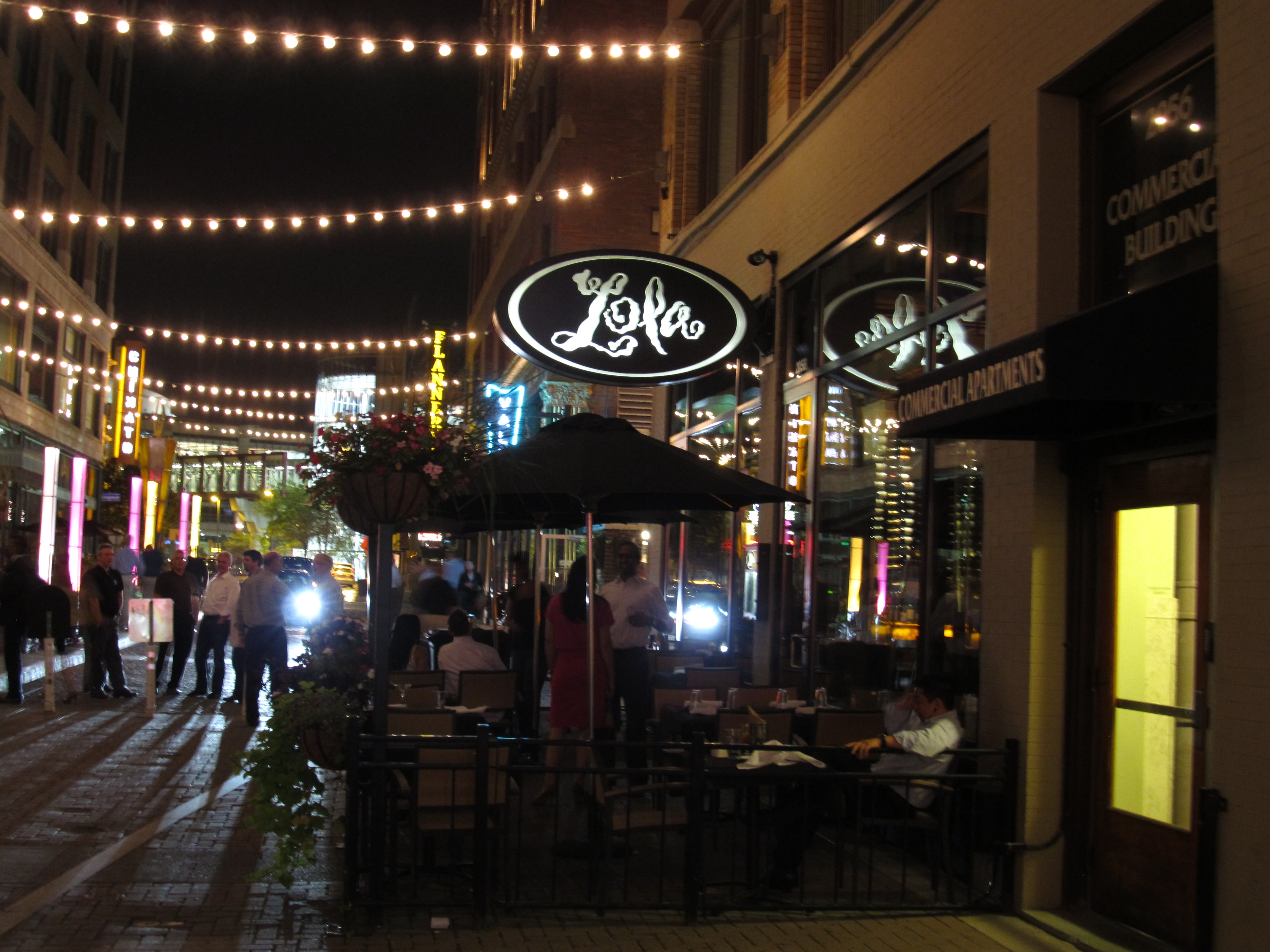The nighttime scene depicts a bustling city area focused around a restaurant named Lola. The oval sign for Lola, with its black background and white cursive text, hangs prominently on the side of the building, illuminated against the night sky. Strands of decorative lights crisscross above the street, casting a warm glow over the area and complementing the street's brick pathway. On the left and right, additional buildings, likely restaurants or bars, add to the lively atmosphere.

Underneath some umbrellas, several tables are occupied by diners. In the lower right-hand corner, a man in a long-sleeved white work shirt, complete with a watch, is leisurely sitting at a table with a linen napkin spread out in front of him. His relaxed posture, with one leg crossed over the other, suggests he is enjoying a casual evening out. Nearby, groups of people are seen standing and conversing in the street, some holding shopping bags and drinks.

Under an awning adorned with baskets of flowers, more people are gathered, reflecting the light shining through the glass windows behind them. The overall ambiance is vibrant and inviting, capturing the essence of a lively urban night scene.